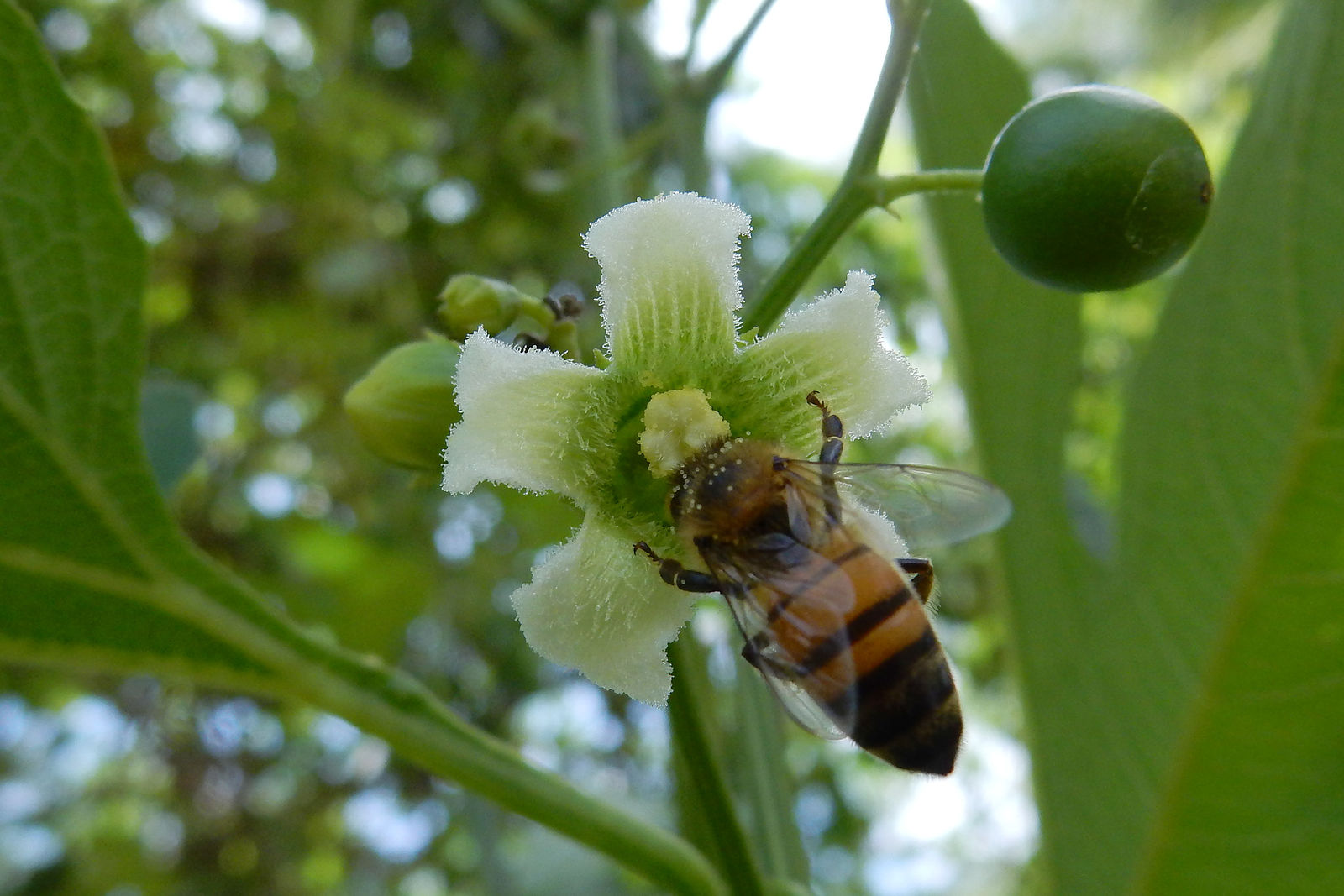This captivating macro close-up photograph showcases a bee diligently pollinating a flower. The bee, with visible pollen dust on its head, is engrossed in gathering nectar from the flower, which features a green center and white-tipped petals. The bee’s front legs are touching the flower as it hovers at an angle, from the left to the right. The detailed shot reveals a green, circular fruit, possibly a lemon or lime, growing above the bee. The background is artfully blurred, highlighting the sharp focus on the bee and the flower, with hints of trees and green vegetation in soft focus.